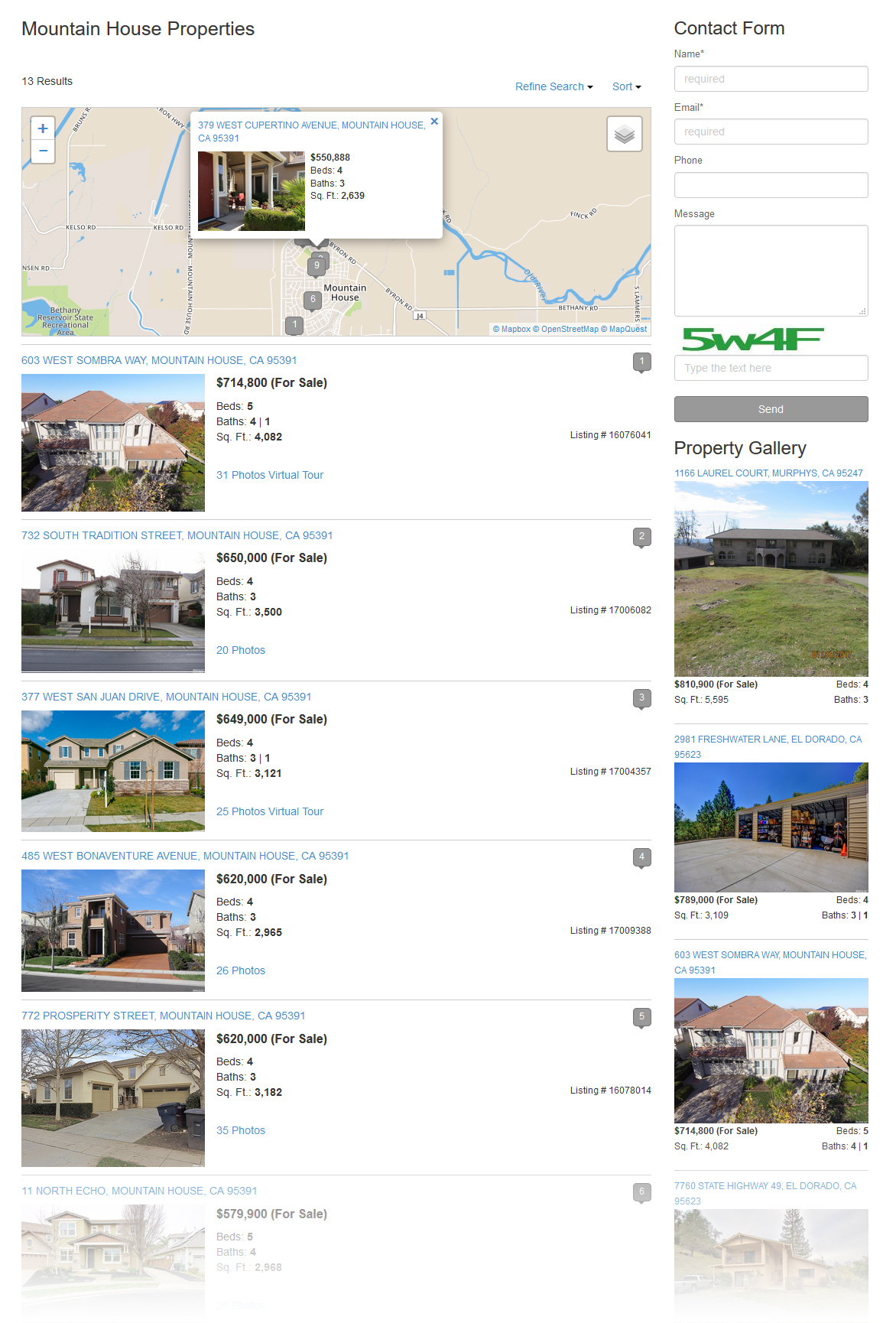This image showcases a property search page, likely focused on mountain houses. At the top of the page, there are 13 search results displayed, with options to refine the search and sort the listings. The page features a series of drop-down menus and hyperlinks accompanied by down-select arrows. 

A contact form is positioned on the page, containing fields for name, email, phone number, and message. The name and email fields have "required" noted in light gray text, and the message box is larger than the other input fields. Below the contact form, there is a captcha code entry box labeled "5W4F," followed by a "Send" button.

The property gallery showcases four images of homes, with the top image being slightly larger and the last image at the bottom fading out into a gradient effect. 

On the left side of the page, beneath a map, there is a section titled "Mountain House Properties," listing six homes. Each listing includes a picture to the left, a value, and a question mark icon at the top right of the box. These listings are separated by light gray horizontal lines, with the bottom listing also fading into a gradient.